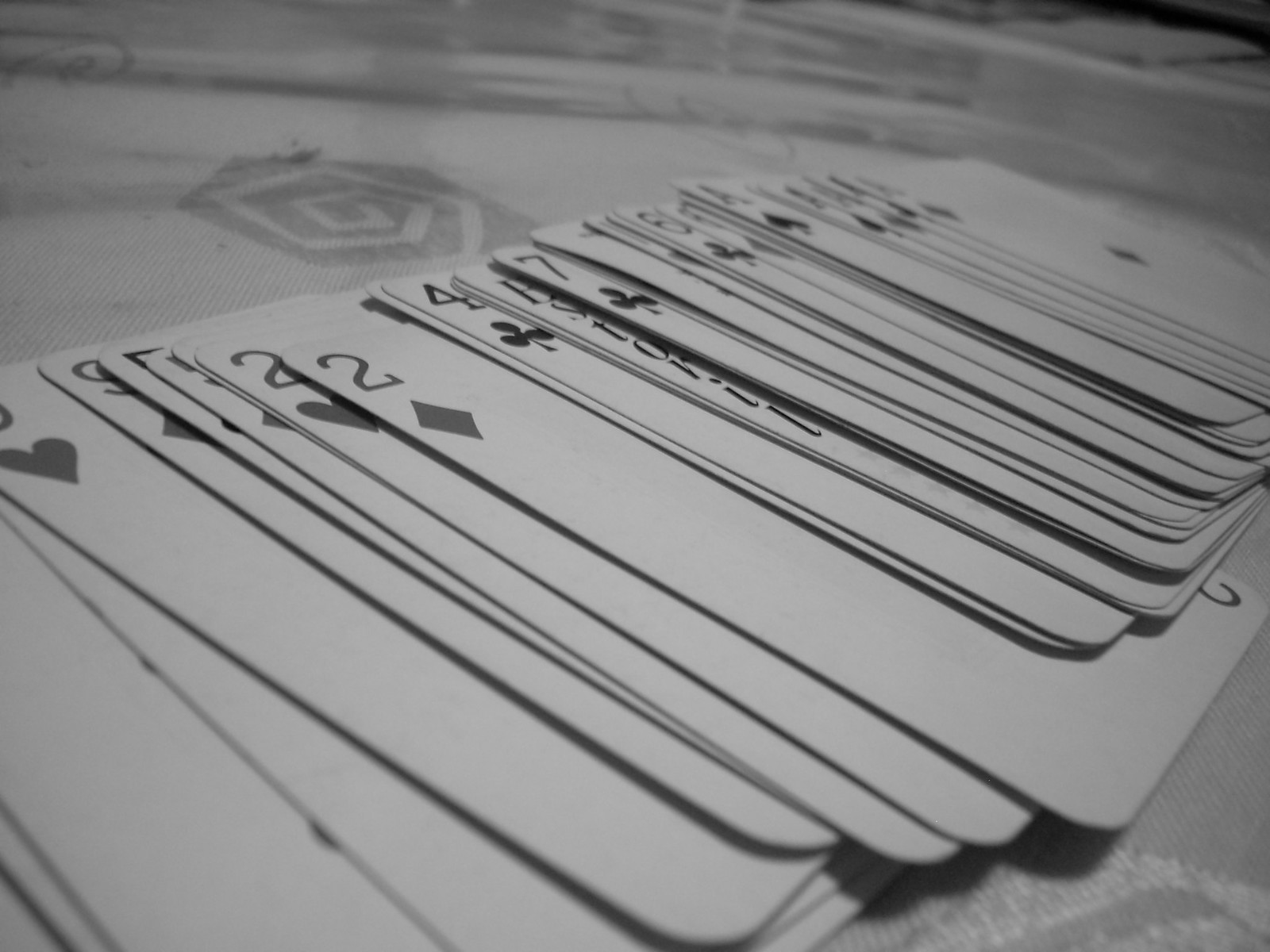This black and white, high-quality landscape image captures a dynamic arrangement of playing cards, artfully scattered in a diagonal formation from the bottom left corner to the top right corner. The cards appear to have been casually spread out, creating an overlapping pattern. The sharp, detailed focus on the lower left reveals cards in excellent condition, starting with a heart, followed by a discernible nine of diamonds. Moving further towards the top right, the cards gradually blur, reducing in clarity and making specific identification difficult beyond a certain point. Among the visible cards are a two of hearts, two of diamonds, four of clubs, a joker, and a seven of clubs. An estimated fifteen more cards continue beyond this visible sequence but fade into the blurred background. The underlying surface is a tablecloth with a linen-like texture, adding to the tactile quality of the composition.